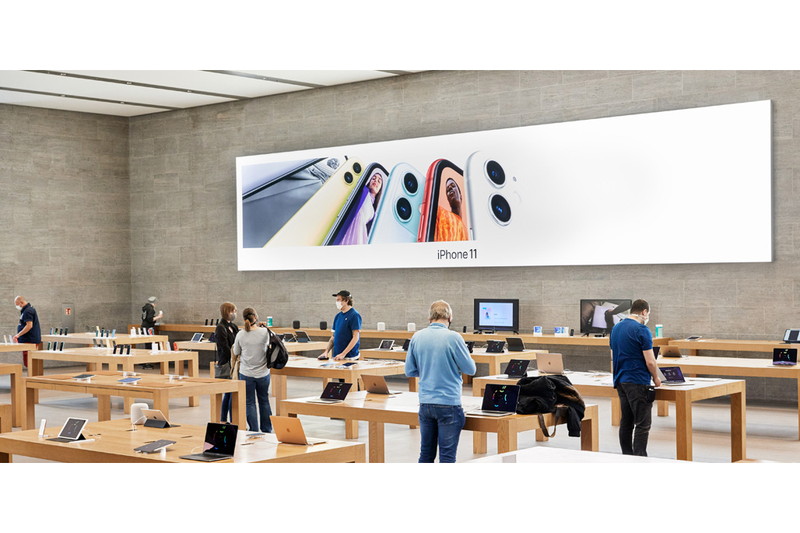This image shows the interior of an Apple Store, highlighting its minimalistic and streamlined design. The store's walls are gray, resembling cinder blocks, while the ceiling is white with exposed gray beams. Dominating the front of the store is a large rectangular advertisement for the iPhone 11, depicting around five or six different phones—some displaying images, others simply showcasing their cameras. The text "iPhone 11" is prominently placed beneath the displayed phones.

The store is arranged with several tables featuring displays of various Apple products, including phones and computers. Patrons, all wearing masks due to COVID-19, are scattered throughout the store, maintaining a safe distance from one another. Individuals are seen trying out products and exploring features independently, with minimal interaction. One notable scene includes a man conversing with two women from afar. Among the shoppers, most are men; one man, in particular, has placed his bag and coat on a table beside the product he is examining. The overall atmosphere of the store is calm and observant, adapted to current health guidelines.